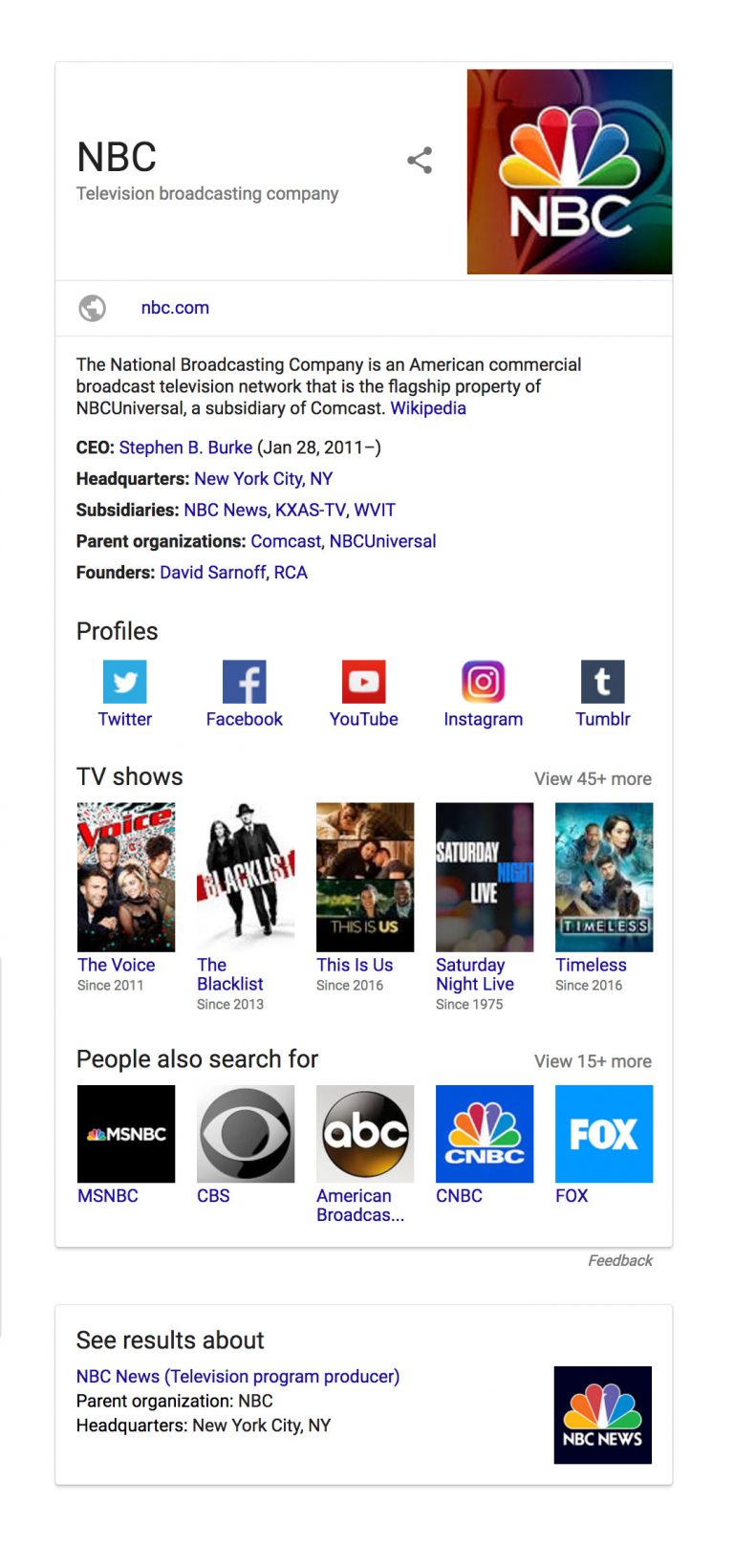The image depicts a screenshot from a smartphone display, showcasing a largely white background with significant information presented in a neatly organized manner. At the top of the image, there's a horizontal line, below which the letters "NBC" appear prominently in large, bold, capitalized text, albeit darker in shade rather than in font weight. Beneath the "NBC" logo, the phrase "Television Broadcasting Company" is displayed, offering clarification, possibly for those unfamiliar with the acronym.

To the right of this, an unconnected triangle symbol is present, its exact meaning not immediately clear. Adjacent to this, the well-known NBC peacock logo is featured, displaying a spectrum of vibrant colors in its feathers.

Further down, the smaller text “NBC.com” is visible, indicating the network’s website. Below this, a detailed definition from Wikipedia outlines that NBC stands for the National Broadcasting Company, an American commercial broadcast television network, serving as the flagship property of NBCUniversal, a subsidiary of Comcast. Additional information from Wikipedia specifies the CEO as Stephen Burke and notes the headquarters are located in New York, New York. It also lists subsidiaries including NBC News and several radio and television stations. The parent organizations are identified as Comcast and NBCUniversal, with founders David Sarnoff and RCA.

The image further includes references to the network's social media profiles on platforms such as Twitter, Facebook, YouTube, Instagram, and Tumblr. A section highlights some of NBC’s famous TV shows and suggests related searches for ABC, MSNBC, CNBC, and Fox, indicating a comparison or exploration of similar networks. The image concludes by hinting at additional results available beneath the provided information.